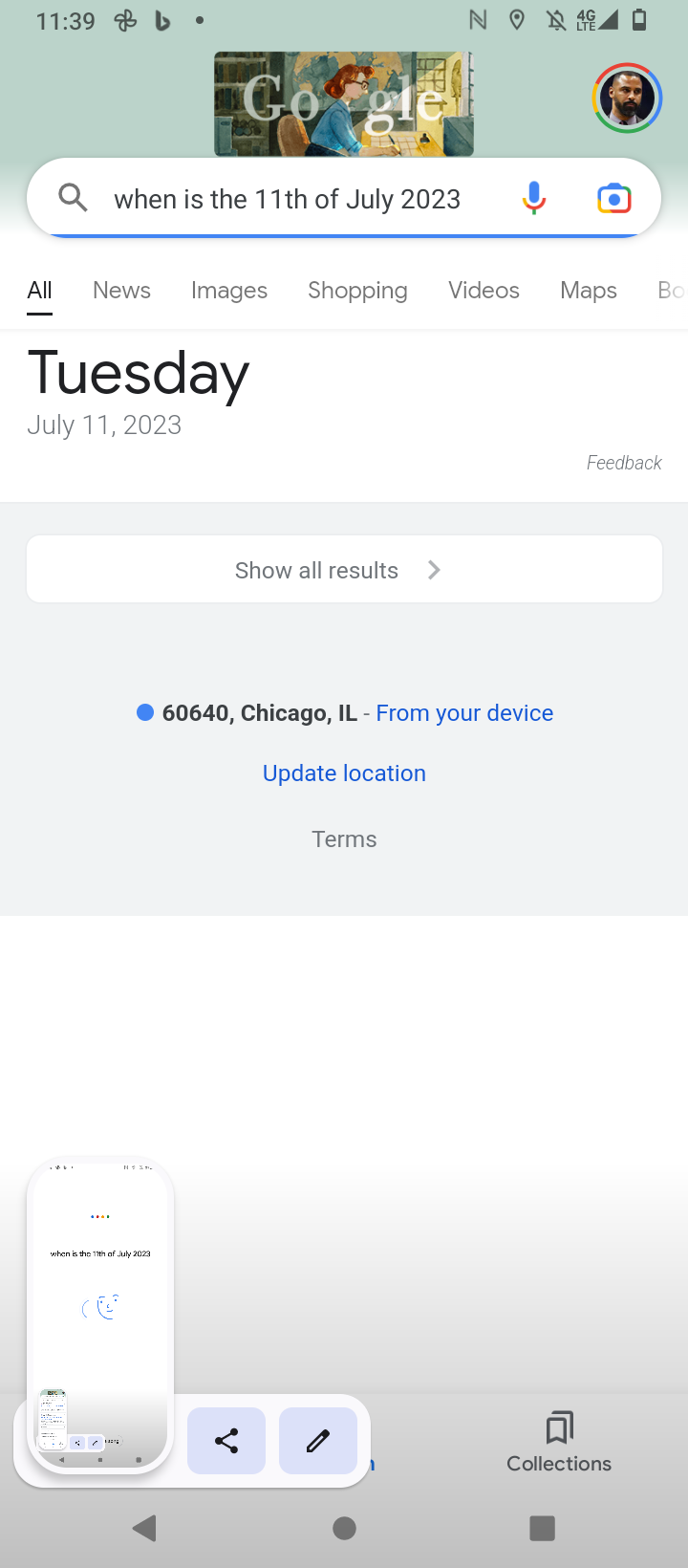The image depicts a smartphone lock screen displaying the date, Tuesday, July 11th, 2023. At the top, there is a green notification bar with a Google search query asking, "When is the 11th of July 2023?" The answer, displayed prominently below, confirms the date as Tuesday, July 11th, 2023. In the top right corner, there is a recognizable icon indicating the user is in Chicago, Illinois, with a location reading "60640" sourced from the device. The status bar at the top of the screen shows standard Android icons, including battery, signal strength, and Wi-Fi indicators. The bottom portion of the screen features icons associated with a phone editing software, suggesting the presence of an app for customizing or editing phone settings or media.